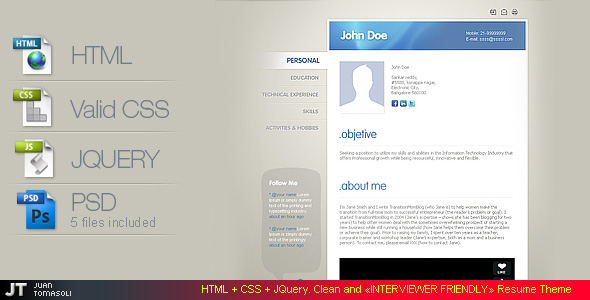This image features the setup screen of a query website, displaying a variety of detailed elements and sections. The website sports a muted gray background with a multicolored bar running along the bottom. On the left-hand side of the screen, an HTML icon is prominently displayed, accompanied by the text "HTML" in a darker shade of gray, emphasizing its importance.

Adjacent to this is a CSS banner, featuring green with white font and a small, recognizable CSS-related logo. This section is labeled "Valid CSS" in gray font, ensuring users that the CSS code adheres to standards. Below this, there is a green box with white letters that spell "JS," indicating a jQuery component.

The final item in this list is presented in a blue bar with an accompanying blue icon and black font, labeled "PSD." This section notes that "5 files included," serving as a counter for the involved files.

Centrally positioned, there's a narrow bar designated for entering personal information. This area is streamlined for user input, facilitating the process of populating the site with individual data.

On the right-hand side, the layout preview for a social media thumbnail site is displayed, giving users a clear visual representation of the final setup. The combination of these elements outlines the comprehensive and user-friendly interface of the query website setup screen.